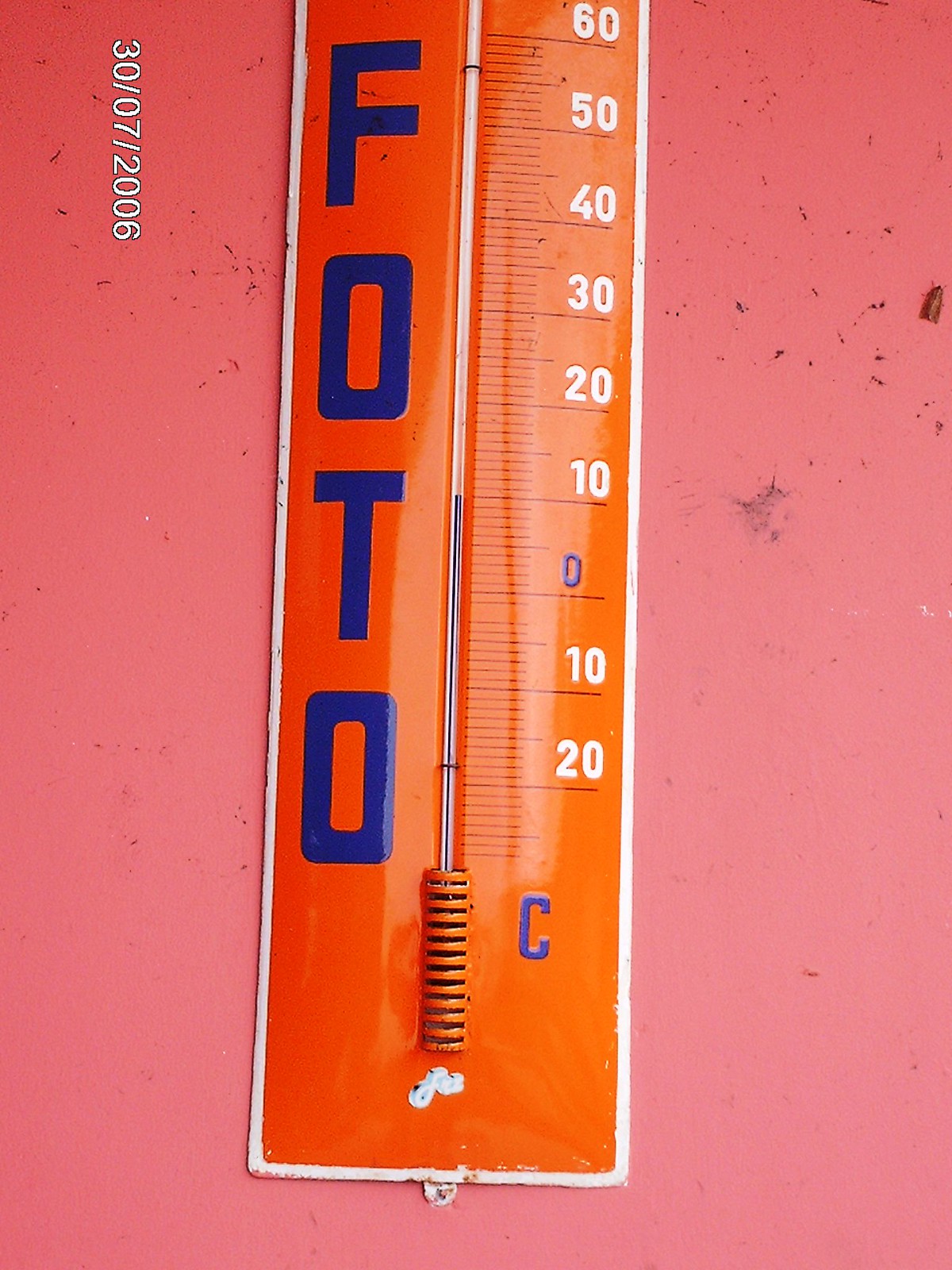This detailed image showcases a close-up view of a food thermometer affixed to a red, possibly scratched, wall. The vibrant red surface features several marks and scratches, along with a date inscribed vertically on the left side: "30-07-2006", requiring the viewer to turn the phone sideways to read it clearly.

The thermometer itself has an orange background with the word "FOTO" prominently displayed in large blue letters, arranged vertically. The temperature scale is measured in Celsius, indicated by a blue 'C'. The scale on the right side starts with blue for zero degrees and continues in white for both the negative range (marked -10 and -20) and positive range, clearly labelled from 10 up to 60 degrees.

The current temperature reading on the thermometer is marked by a blue line, which is precisely at 10 degrees Celsius. Surrounding the thermometer is a thin white frame, which appears to be nailed to the red wall, reinforcing its vertical positioning. The meticulous details in the frame, scratches, and the alignment suggest that this thermometer is securely installed for regular use or display.